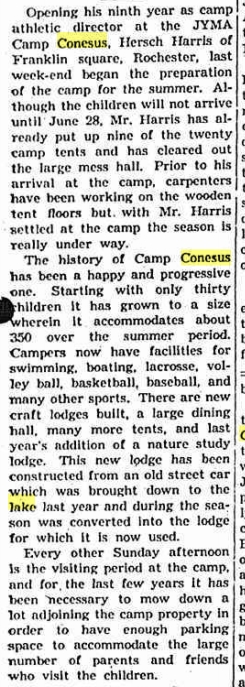This image shows a newspaper clipping featuring black text against a white background, with certain sections highlighted in yellow. It details the start of Hirsch Harris's ninth year as the camp athletic director at JYMA Camp Conesus in Franklin Square, Rochester. Last weekend, Harris began preparing for the summer season even though the children won't arrive until June 28. By this point, he has already erected nine out of the 20 camp tents and has cleared out the large mess hall. Before Harris's arrival, carpenters were busy working on the wooden tent floors, but now that he has settled in, the camp season is officially underway. 

Camp Conesus boasts a happy and progressive history, growing from initially serving 30 children to now accommodating about 350 campers over the summer. The camp offers a wide array of facilities including swimming, boating, lacrosse, volleyball, basketball, baseball, and many other sports. Recent additions to the camp include new craft lodges, an expansive dining hall, and increased numbers of tents. Notably, last year saw the introduction of a nature study lodge, ingeniously repurposed from an old streetcar transported to the lake. 

Every other Sunday afternoon is a designated visiting period when parents and friends come to visit the children. The influx of visitors has necessitated mowing down an adjoining lot to provide sufficient parking space.